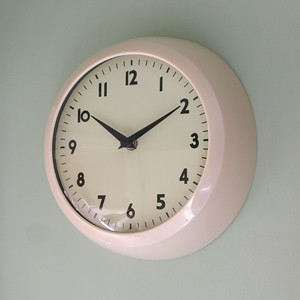The image is a color photograph of a simple, no-frills clock mounted on a gray wall. The circular metal clock features a pink rim and an off-white face. Its black hands, lacking a second hand, and black numbers clearly display the time as 10:10. The clock's glass face reflects some light, causing noticeable bright spots on its surface and along the bottom right-hand corner, suggesting the presence of a light source in the room. There's a faint shadow cast by the clock onto the wall, enhancing its dimensional appearance. Overall, the clock is straightforward, without any additional designs or maker's name visible.